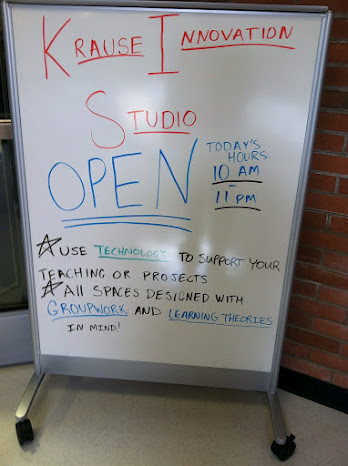The image features a large vertical whiteboard sign with a silver frame and black casters at the base, allowing it to roll. The board stands against a red brick wall, and nearby, there's a silver-framed window. The floor beneath it appears off-white, possibly a basic terrazzo surface. The whiteboard itself displays colorful and detailed text. At the top, in red writing, it reads "Krause Innovation Studio." Below that, in large blue letters, the word "Open" is written and underlined twice. The schedule "Today's hours: 10 a.m." and "11 p.m." is noted in smaller blue letters, each underlined in black. There are stars highlighting additional information: "Use technology to support your teaching or projects," with "technology" written in turquoise and underlined. Another star indicates, "All space is designed with group work and learning theories in mind," with "group work" and "learning theories" in blue and underlined.